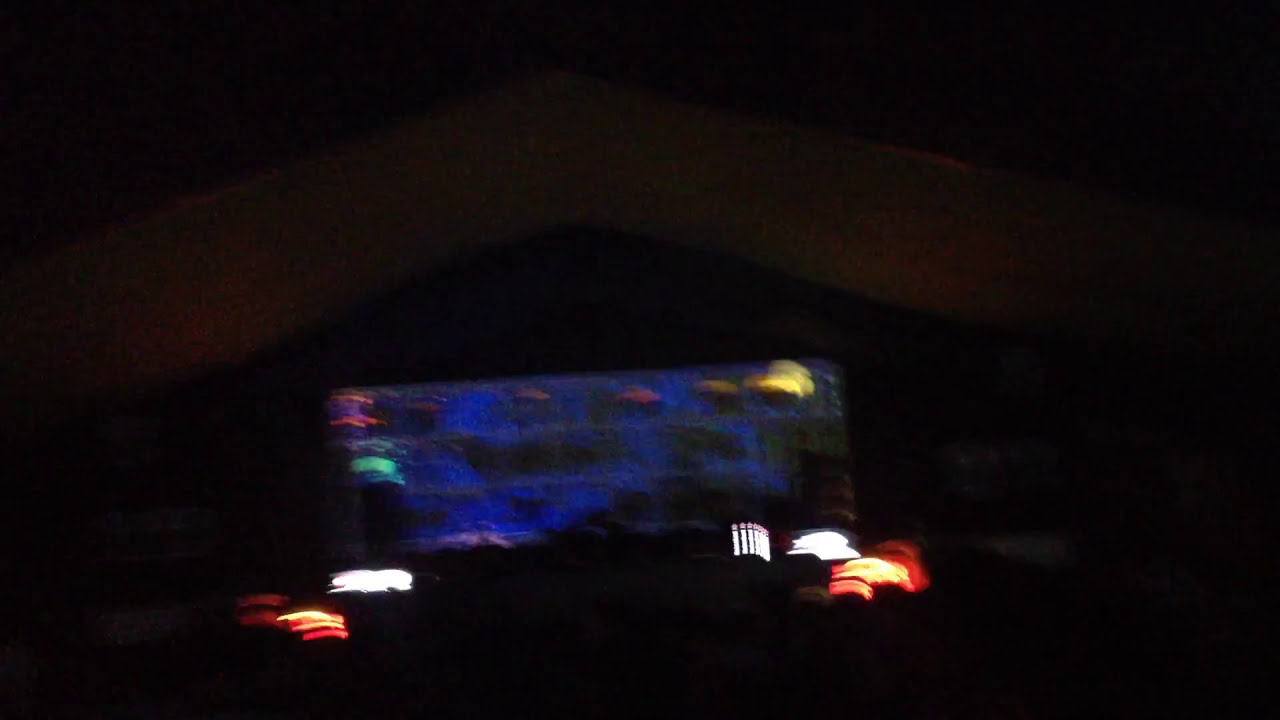The image is an extremely blurry nighttime photograph, likely taken with an old or shaking camera, making it difficult to discern clear features. The entire background is predominantly black, emphasizing a sense of darkness around the central subject. Front and center appears to be a multi-story building, potentially a hotel, illuminated with shades of green, red, and yellow lights, giving it an almost spectral appearance. The structure, possibly up to five stories high, presents an array of blurry lights: on the left-hand corner, there's a red light positioned just above a green one, while the far right-hand corner displays a series of yellow lights. Adding to the confusion are horizontal blue rectangular sections that might be windows or a screen, sectioned into smaller squares, giving a grid-like effect. In front of the building, blurred red, orange, and yellow streaks of light, possibly from passing vehicles, mirror each other on either side. No discernible text or people are visible in the image, which features light trails suggesting motion, blending into the dark backdrop.